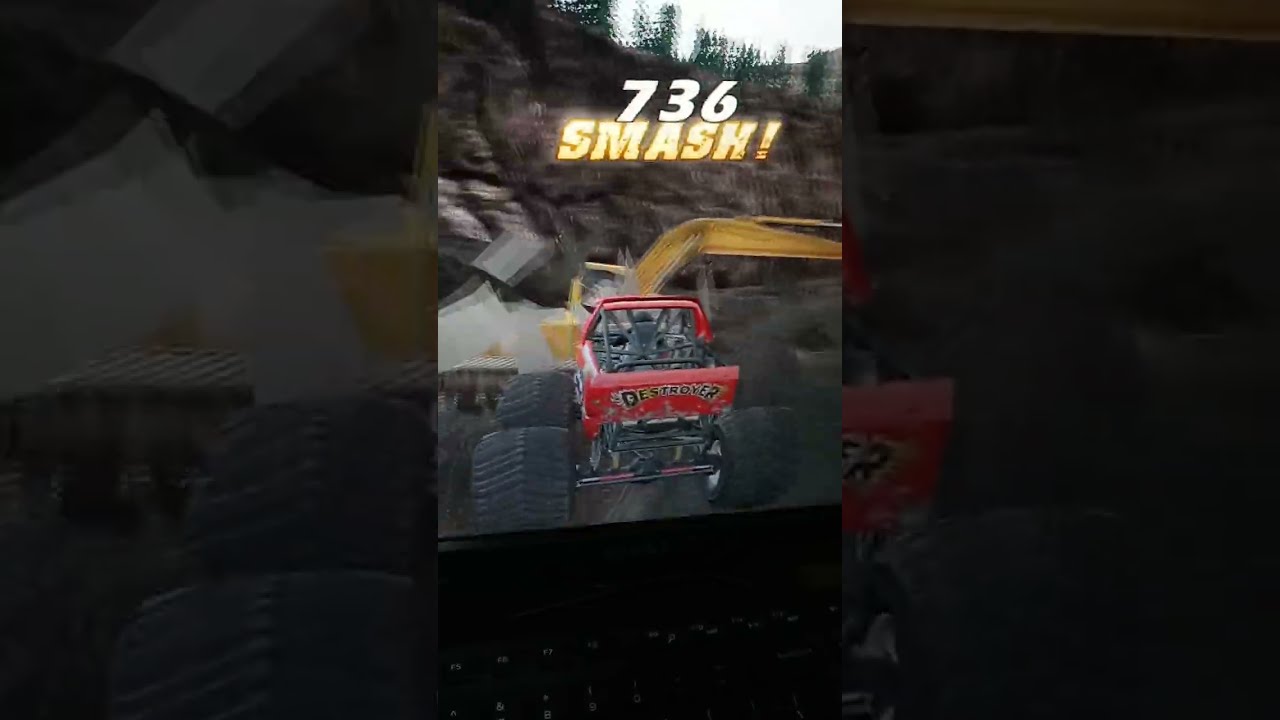The image depicts a dynamic scene with a red monster truck prominently positioned in the foreground. The truck, adorned with a black roll cage and mammoth tires extending from visible axles, bears the bold inscription "DESTROYER" in black and yellow on its tailgate. Above the truck, the large white bubble numbers "736" and the word "SMASH!" in vibrant yellow command attention. These letters hover over a background dominated by a mountainside, with brown rocky terrain and a sparse collection of evergreen trees atop the bluff. The background scene is blurred, providing a stark contrast to the sharply focused truck and its details. The photograph appears to capture an outdoor setting, possibly a junkyard or an area strewn with debris. Despite the indistinct nature of the debris, a yellow streak reminiscent of an excavator’s arm can be seen extending from the front of the truck. The sky is visible in the upper right corner, indicating the daylight setting, with a faint outline of a structure against the blue. The scene encapsulates a sense of motion and chaos, epitomized by the monstrous vehicle seemingly amidst a thrilling clash with the surrounding terrain.